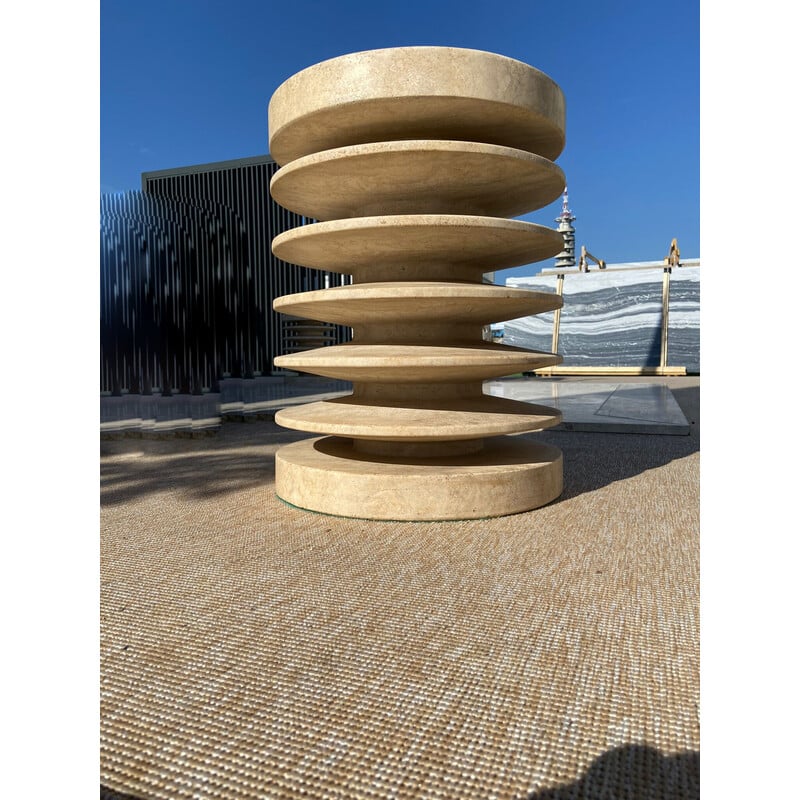The image showcases a large outdoor sculpture, prominently featuring a cylindrical, screw-like form with spirals or alternating plates in a tan, wooden texture. The sculpture is heavier at the top and bottom, creating a balanced base, and it rests on a surface that appears to be a tan carpet. The backdrop reveals a bright, sunny day with a clear blue sky devoid of clouds. To the right of the sculpture, there's a marble wall and a secondary gold sculpture, while on the left, there's a building that appears black and potentially distorted in the image, possibly with a fence-like structure. The entire setting is brightly lit by the sun, highlighting the rough texture and intricate design of the sculpture.